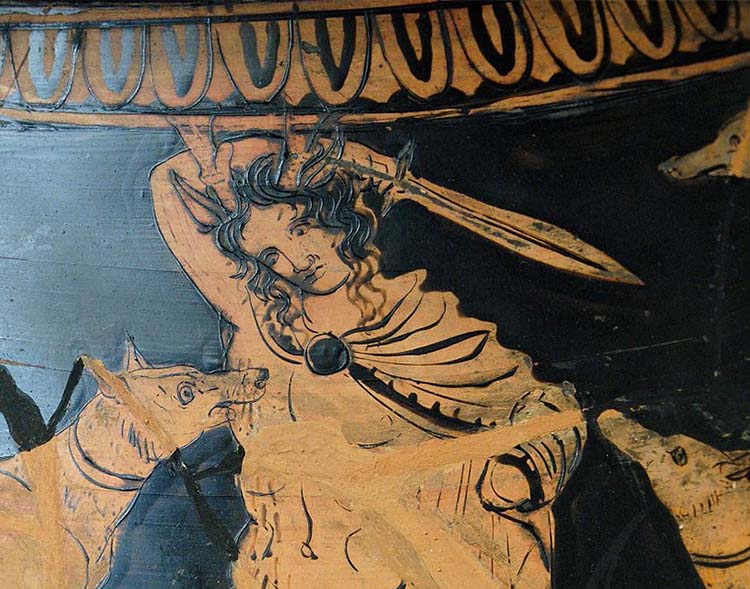The image showcases a detailed art piece that appears to be either an engraving or a painting on a wooden or pottery surface. The background is black, with the artwork rendered in a goldish-beige or brown hue, emphasizing intricate line workings. Central to the composition is an androgynous figure with long hair, holding a sword aloft in a battle-ready stance. The figure exhibits both feminine and masculine traits, with facial features more closely resembling a male. Surrounding this central figure are two wolves. One wolf is aggressively biting into the figure's chest or armpit, while the head of another wolf is visible from the right side of the image. The scene's backdrop includes a series of V-shaped banners or decorative symbols extending from left to right at the top of the image, possibly indicating the artwork's location on the curved surface of a vase or similar object. The shiny surface with light reflections suggests the use of black paint or ink, enhancing the dramatic contrast and highlighting the detailed craftsmanship of this evocative piece.